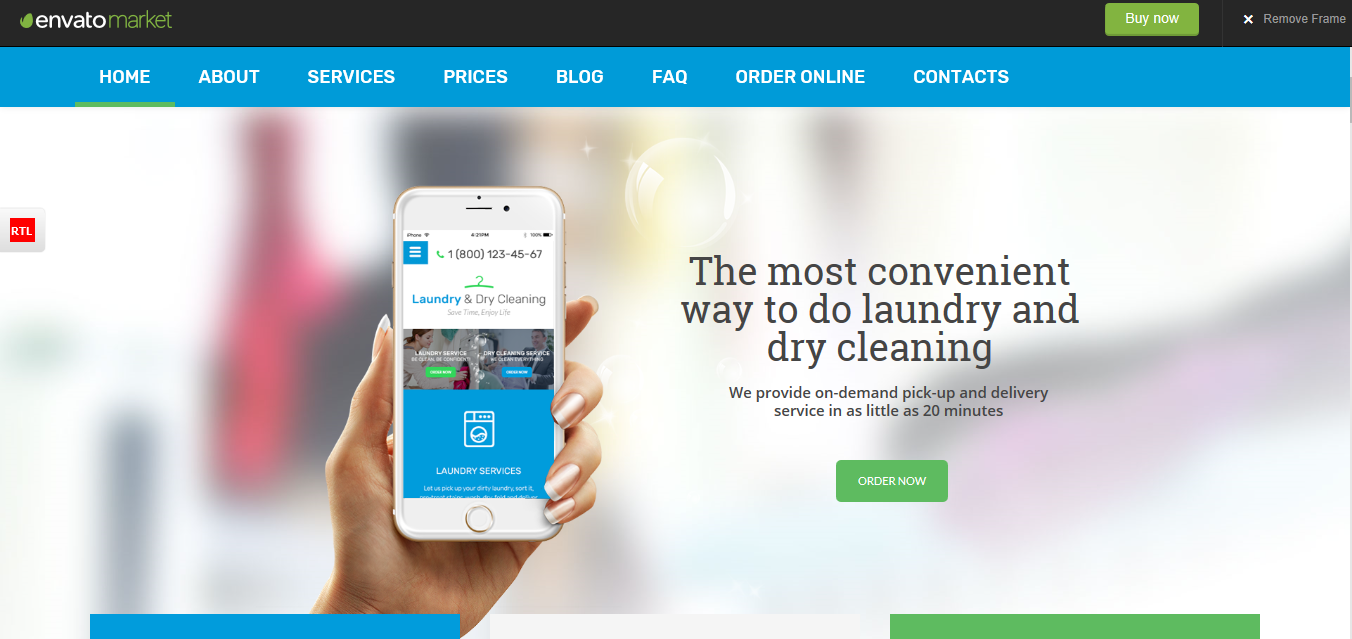The image is a rectangular banner, roughly twice as wide as it is tall. At the top, there is a horizontal black bar occupying approximately 5-10% of the image's height. In the upper left corner of this bar, there is a company logo featuring a green swoosh and the text "Envato" in white. Following this, the text changes to an olive green color, spelling "Market," forming the full company name "Envato Market." Towards the right side of the black bar, there are two elements: a green button with white text reading "Buy Now" and, next to it, a white 'X' followed by gray text that says "Remove Frame."

Below the black bar, a blue horizontal bar spans the width of the image, taking up about 10% of the image's height. This blue bar has a medium hue and contains several menu items written in white capital letters: HOME, ABOUT, SERVICES, PRICES, BLOG, FAQ, ORDER ONLINE, and CONTACT. A green line beneath "HOME" indicates that it is the selected tab.

The majority of the image is occupied by a large banner. On the left third of this banner, a hand is positioned, holding a cell phone. The screen of the cell phone is clearly visible, drawing attention to its display.